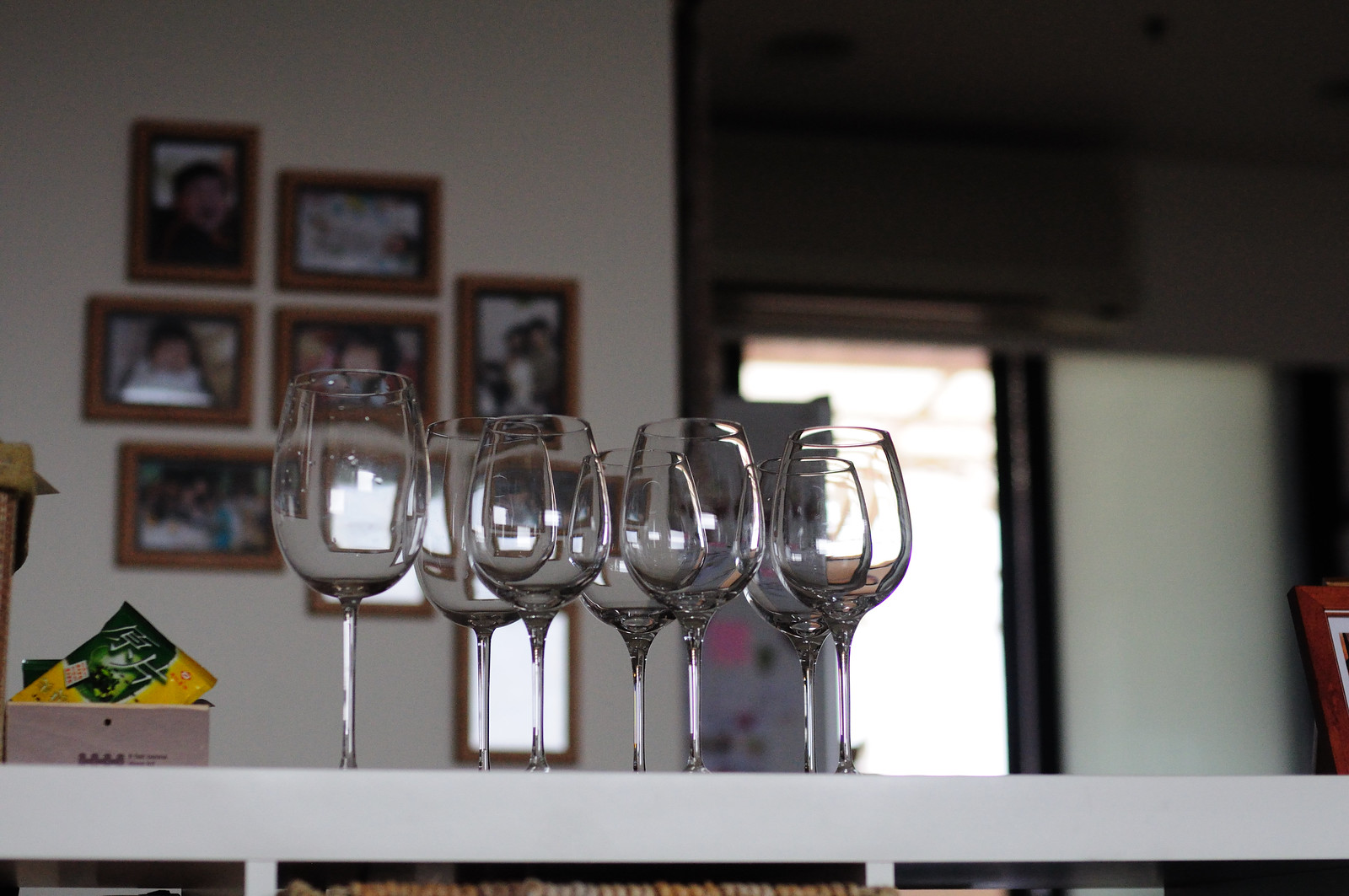The photograph captures a bright indoor scene centered around seven empty, transparent wine glasses of varying sizes positioned on a white countertop. Behind the glasses is a wall adorned with multiple family photos in brown wooden frames, some in portrait and others in landscape format. The reflections of these frames can be seen on the wine glasses. To the left of the glasses, a small yellow bag with green labeling contains seaweed chips. An open sliding door to the right allows daylight to flood the space, indicating it is daytime. Adjacent to the door, a refrigerator covered with magnets and the edge of another wooden picture frame further decorate the scene. Additionally, a box and part of a bookcase are seen at the periphery, contributing to the detailed composition of the room.